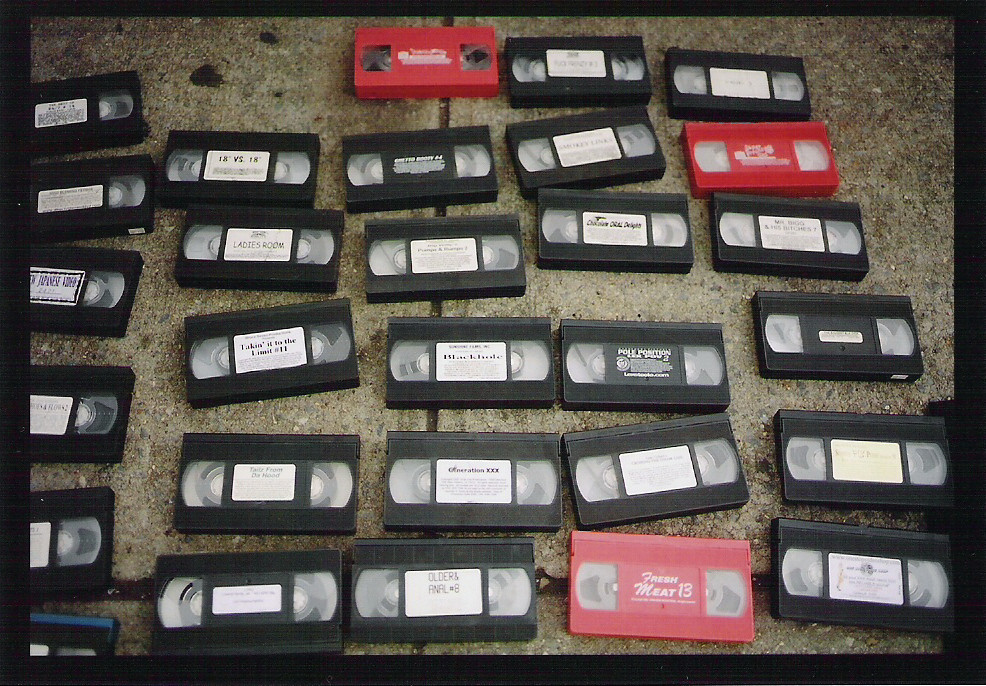This photograph captures a collection of approximately 30 VHS tapes, predominantly black with a few red ones scattered throughout. The tapes, which are out of their cases, are laid out on a slightly dirty cement sidewalk. The arrangement forms a semi-neat grid of five columns and six rows, but the alignment is somewhat irregular. The concrete beneath features visible seams and some moss stains. Notably, one tape in the bottom left corner has a distinctive blue stripe. Several of the visible labels suggest that the tapes are adult films, with titles including "XXX."